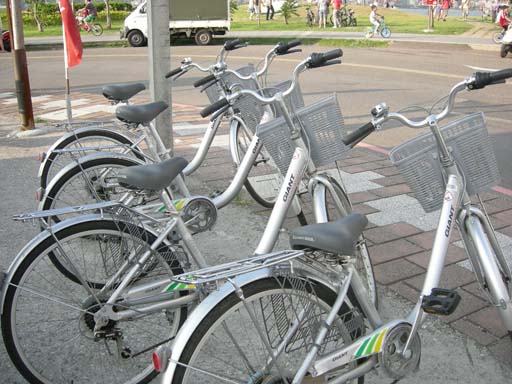The photograph captures a street corner bustling with life on a pleasant day. In the foreground, four identical cruiser bicycles are neatly lined up side-by-side on a cement sidewalk. These bikes are characterized by their sleek, thin frames painted in white. Each bike is equipped with silver wire baskets in the front and chrome fenders with little red taillights at the back. The handlebars are silver with black grips, and they feature silver book racks. Additionally, the bikes have big wheels with silver covers, and they appear to be rental bikes, possibly indicated by green and yellow stripes on the protective sprocket covers and the brand name "Giant."

Beyond the bikes, the street extends, featuring a typical yellow line running down the middle. The street curves to the left, intersecting with another road, possibly hinting at a busy street corner. On the opposite side of the street, there's a park teeming with activity. People can be seen riding bikes, sitting in the grass, and enjoying the green lawn and scenic surroundings. Adding to the urban atmosphere, a box truck is parked at the curb, and the scene is further animated by cars driving up and down the road. The overall setting suggests a vibrant, lively area, possibly in a city, with the park offering a peaceful contrast to the busy street.